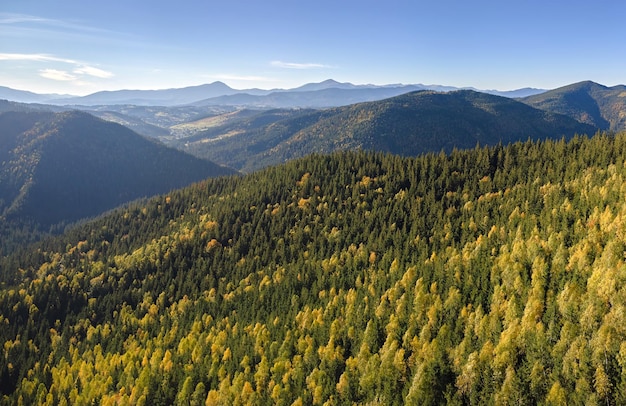The photograph captures an expansive landscape of untouched nature taken from an aerial perspective during the daytime. In the foreground, there is a dense, hilly forest with a canopy of trees that range in color from a yellowish green to a darker green as you move towards the center of the image. The undisturbed trees appear lush and plentiful, highlighting the natural beauty of the area. The mid-ground reveals rolling hills also covered in dense forest with the darker green hues becoming more prominent. Further back, the scene transitions into large, dark-colored mountains topped with vegetation, while a thin white mist adds a mystic quality to the distant background. In the far horizon, the outline of more distant mountain peaks emerges, shrouded in a lighter haze. The sky above is a clear blue on the right side, gradually merging with wispy white clouds toward the left, enhancing the serene and untouched essence of this vast wilderness. No man-made structures or identifying text are present in the image, emphasizing the pure natural landscape.